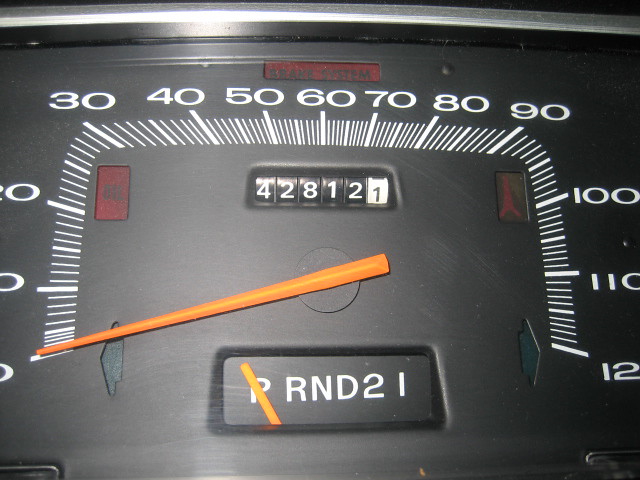The image captures a close-up view of a car's speedometer and gear indicator. The speedometer dial ranges from 0 to 120, likely in miles per hour given the gauge layout common in American vehicles. At the center of the dial, a bright orange hand indicates the current speed, though the exact speed isn't specified in the description.

The car's odometer reads an impressive 428,121 miles, showcasing substantial use. Next to the speedometer, the gear indicator is prominently displayed, denoting the car’s automatic transmission. The gear positions are labeled as P for Park, R for Reverse, N for Neutral, and D for Drive, along with lower gear options marked as 2 and 1. The car is currently in the 'Park' position, as indicated by the red pointer on the gear dial.

This visual layout aids the driver by providing clear, immediate information about both their speed and gear status, enhancing driving safety and convenience by reducing the reliance on the gear lever position alone.